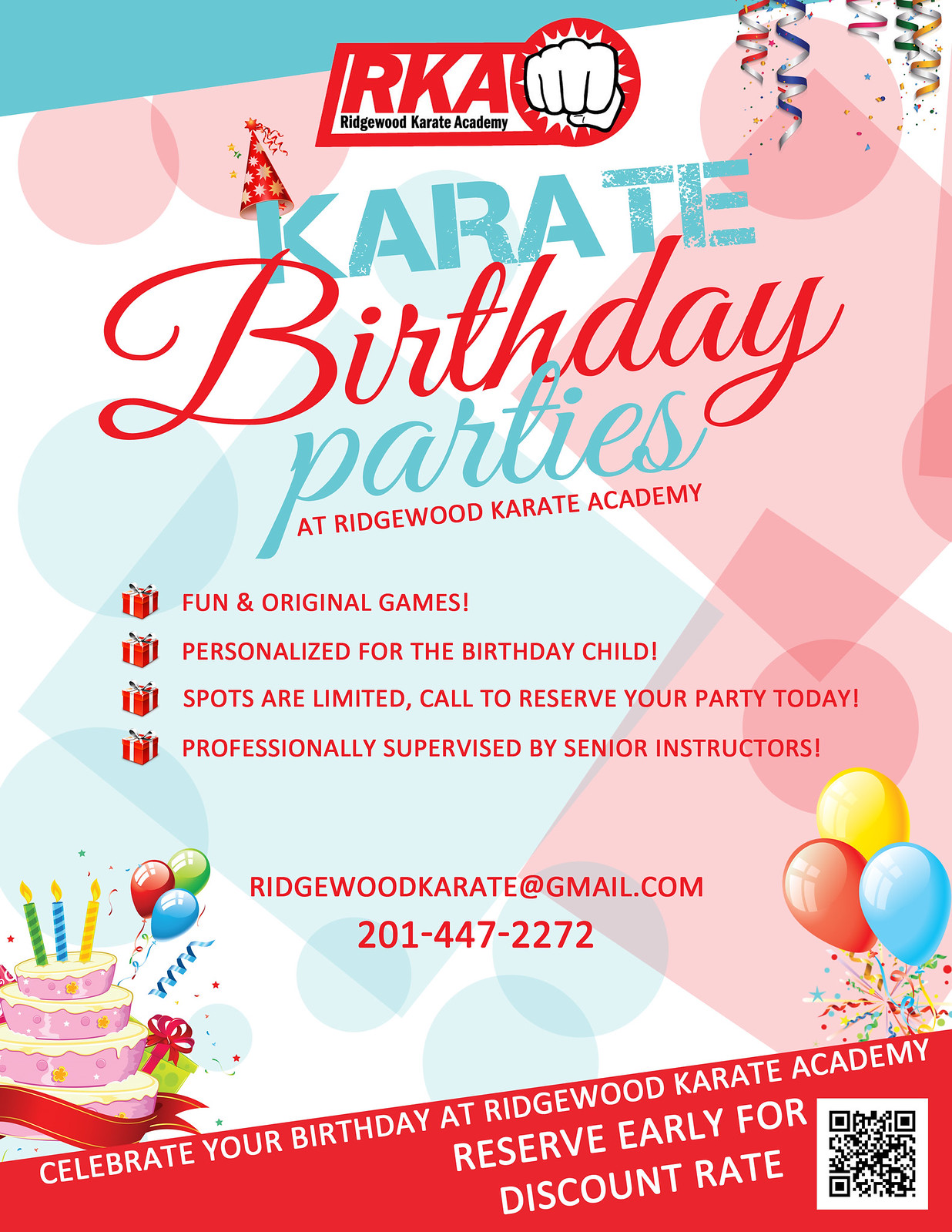The advertisement poster for Ridgewood Karate Academy's Karate Birthday Parties features a bold title at the top, "Karate Birthday Parties at Ridgewood Karate Academy," with the acronym "RKA Ridgewood Karate Academy" and a fist logo directly above it. The words "Karate" and "Parties" are highlighted in blue, while "Birthday" stands out in red; the "K" in "Karate" is adorned with a party hat. Enhancing the festive vibe are four red present emojis, each introducing a new line of text underneath the title: "Fun and Original Games," "Personalized for the Birthday Child," "Spots Are Limited," and "Call to Reserve Your Party Today." It also mentions that the events are "Professionally Supervised by Senior Instructors," followed by contact details, including an email address (ridgewoodkarate@gmail.com) and a phone number (201-447-2272). A red section at the bottom further encourages early booking for a discount, with celebratory visuals like birthday streamers, colorful party balloons, and a cake with candles adorning the left side, while additional balloons and a QR code appear on the right. The background is predominantly white, decorated with pink and blue squares and circles, adding to the cheerful and festive atmosphere.